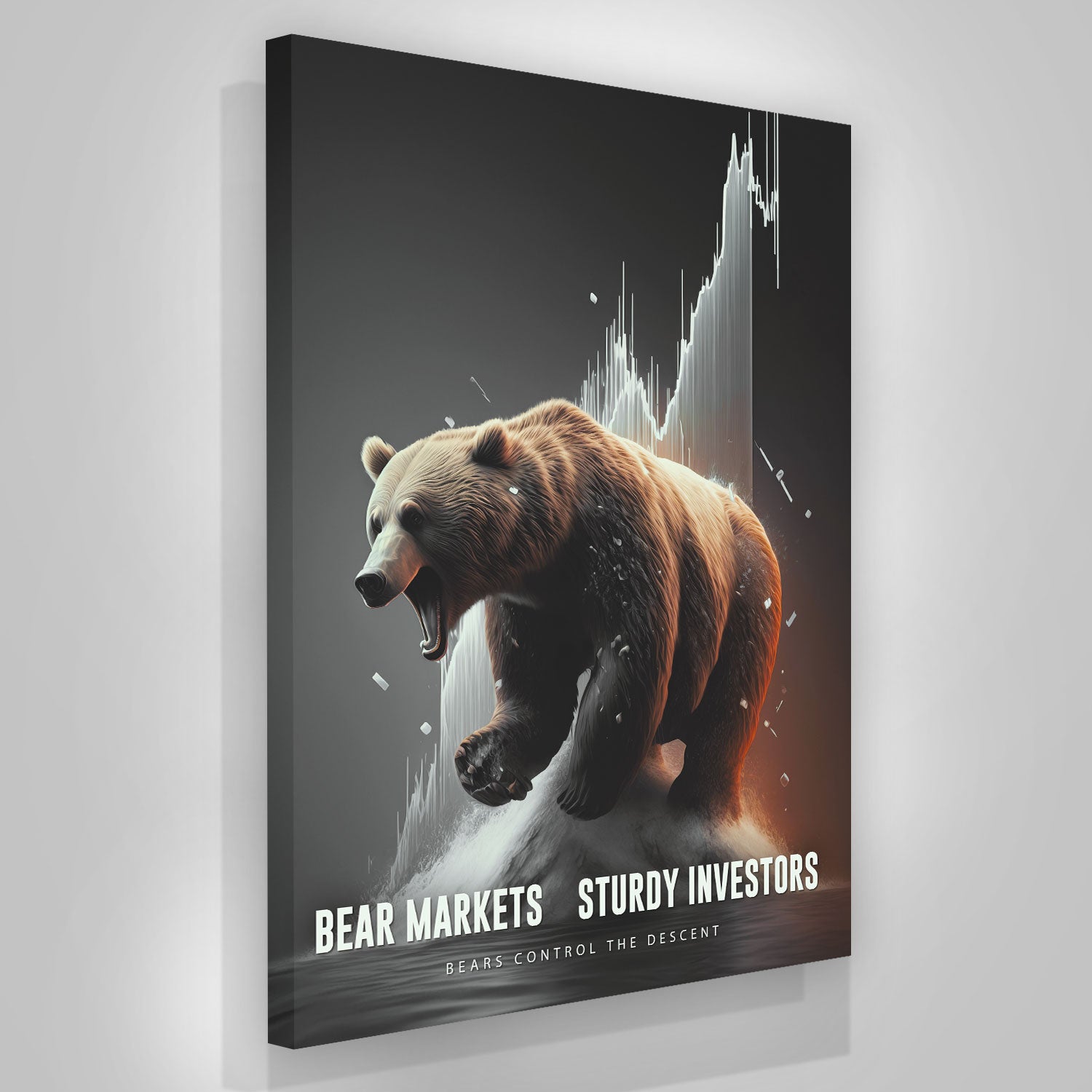The image is a detailed 3D render of a canvas seemingly mounted or hovering just above a wall, casting a shadow for a realistic effect. The canvas depicts an illustration of a large brown bear, mid-jump, with its mouth open wide. The bear is situated on top of a snowy mountain, with splashes of foamy water below, merging seamlessly into the background. The bear's form appears illuminated, with a reddish-orange light from the right and above, accentuating the top and back legs.

Behind the bear is a black-and-white stock market graph, showcasing the peaks and valleys typical of financial candlestick charts. This graph forms part of the backdrop, enhancing the visual complexity of the scene. Beneath the illustrated bear, large white text reads, "Bear Markets" on the left and "Sturdy Investors" on the right, with smaller text stating, "Bears Control the Descent" at the lowest point. The entire scene is dominated by a contrasting black background, with an orange light source infusing the right side of the image, adding depth and intensity to the composition.